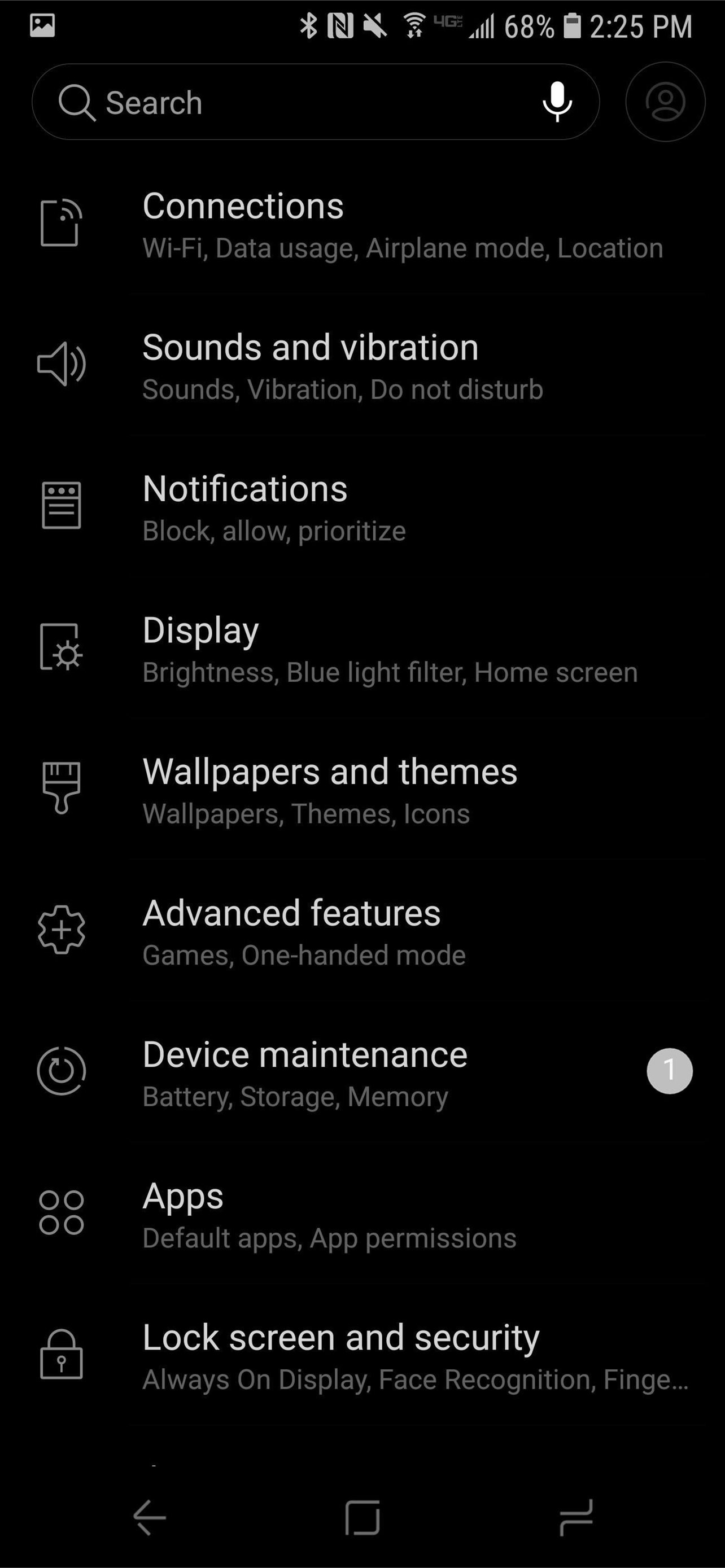The image displays a screenshot taken from a cell phone, where the background of the screen is entirely black. At the top of the screen, various status icons indicate key information: the battery is at 28%, and the current time is 2:25 PM. Below these indicators, there is a search bar. 

On the left side of the screen, a vertical menu is present, displaying a series of icons followed by their corresponding labels in white text. The topmost icon resembles a piece of paper and is labeled "Connections." Moving down the list, a speaker icon is labeled "Sounds and Vibration." A calculator icon follows, labeled "Notifications," and beneath it, an icon showing a piece of paper with a sun is labeled "Display." Continuing down, a paintbrush icon says "Wallpapers and Themes," followed by a gear icon labeled "Advanced Features." 

Further down the menu, a circle icon with another circle inside it is marked as "Device Maintenance," which notably has a gray circle with the number one beside it, indicating a notification or alert. The menu continues with four circles representing "Apps," and a lock icon at the bottom labeled "Lock Screen and Security." 

Overall, the image captures a detailed view of a phone's settings menu, providing a clear look at the various sections available for user configuration.